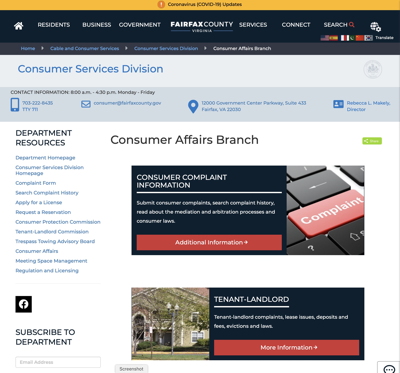This image is a cropped, low-resolution screenshot of a website, likely viewed on a desktop or tablet. At the top of the webpage, there's a yellowish-orange banner with a coronavirus COVID-19 updates notice, which typically redirects users to more information when clicked. Below it, a navy blue banner displays the text "Fairfax County" prominently in white at the center. This banner includes clickable elements labeled: "Residents," "Business," "Government," "Services," "Connect," and "Search," the last of which features a red search icon.

Further down, two light blue banners are visible. The first one reads "Consumer Services Division" in blue text. The second banner's text is small and difficult to decipher but includes icons suggesting communication methods: a cell phone, an envelope (mail), a map pin typically seen on Google Maps, and an icon resembling an ID card.

Underneath these banners, "Consumer Affairs Branch" is written on a white background. To the left, "Department Resources" is listed with approximately 10-11 blue hyperlinks underneath it. The central focus of the page is titled "Consumer Complaint Information," beside which is an image of a keyboard where the Enter key has been replaced with a large, red button labeled "Complaint."